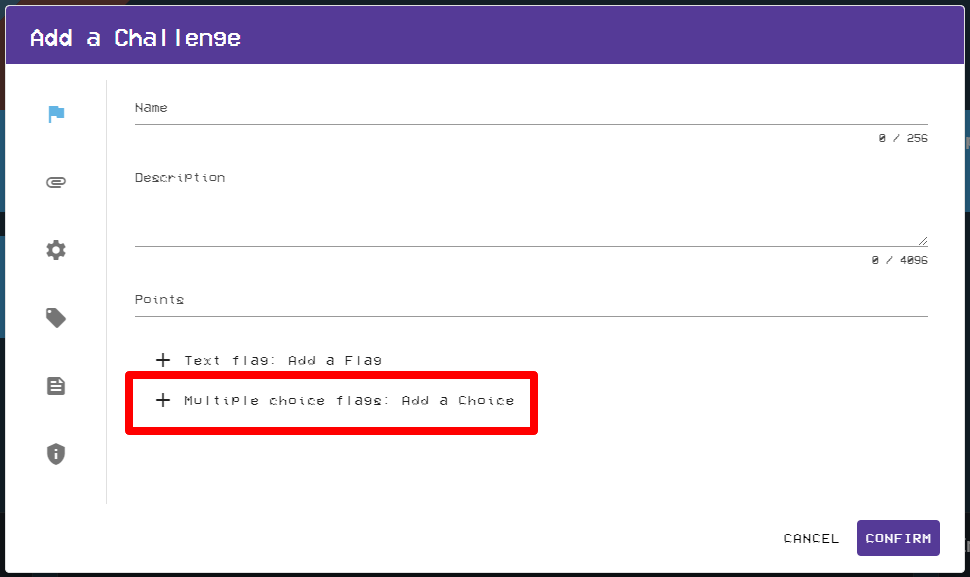The image depicts a vintage computer application's screenshot, showcasing a rectangular dialog box. At the top, a navy blue horizontal bar bears the white text "Add a Challenge." The main area below this header features a white, slightly off-white, grayish background. On the left side, there are six icons arranged vertically; most of them are gray, representing various symbols including a paperclip, gear, tag, piece of paper, and a security badge. The top icon, shaped like a flag, is highlighted in blue. 

On the right side of the dialog box, several input fields are displayed, labeled "Name," "Description," and "Points." Below these fields, there are two options, each with a plus sign preceding some text. The first option reads "Text Flag: Add a flag," while the second reads "Multiple Choice Flags: Add a choice," the latter being particularly emphasized with a bold red rectangle around it.

At the bottom right corner of the dialog box, the options "Cancel" and "Confirm" are available for user interaction.